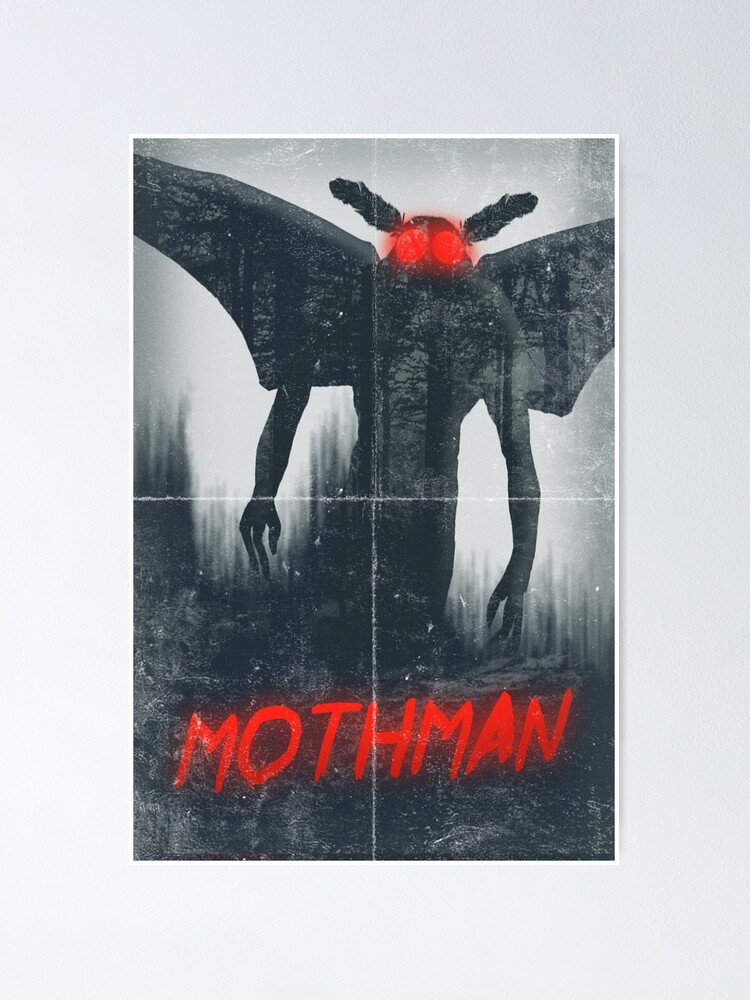The image is a detailed, atmospheric poster for a fictitious figure named Mothman, set against a grayish-white background with visible creases indicating it has been folded into four quarters. The main subject of the poster is a sinister, black silhouette of a creature with a human-like torso and arms, but distinctively moth-like features. These features include large, moth-shaped wings, glowing red eyes, and prominent antennae on its head. The figure's hands are notably unusual, with only a thumb and two extraordinarily long fingers that almost touch the plant life below. In the lower part of the poster, the name "Mothman" is prominently displayed in bold, red letters against a darker background. The bottom part of the image also features gray and black tones, along with hints of plant life and grass. The figure's haunting, insectoid presence against the minimalist background creates an eerie and captivating visual.